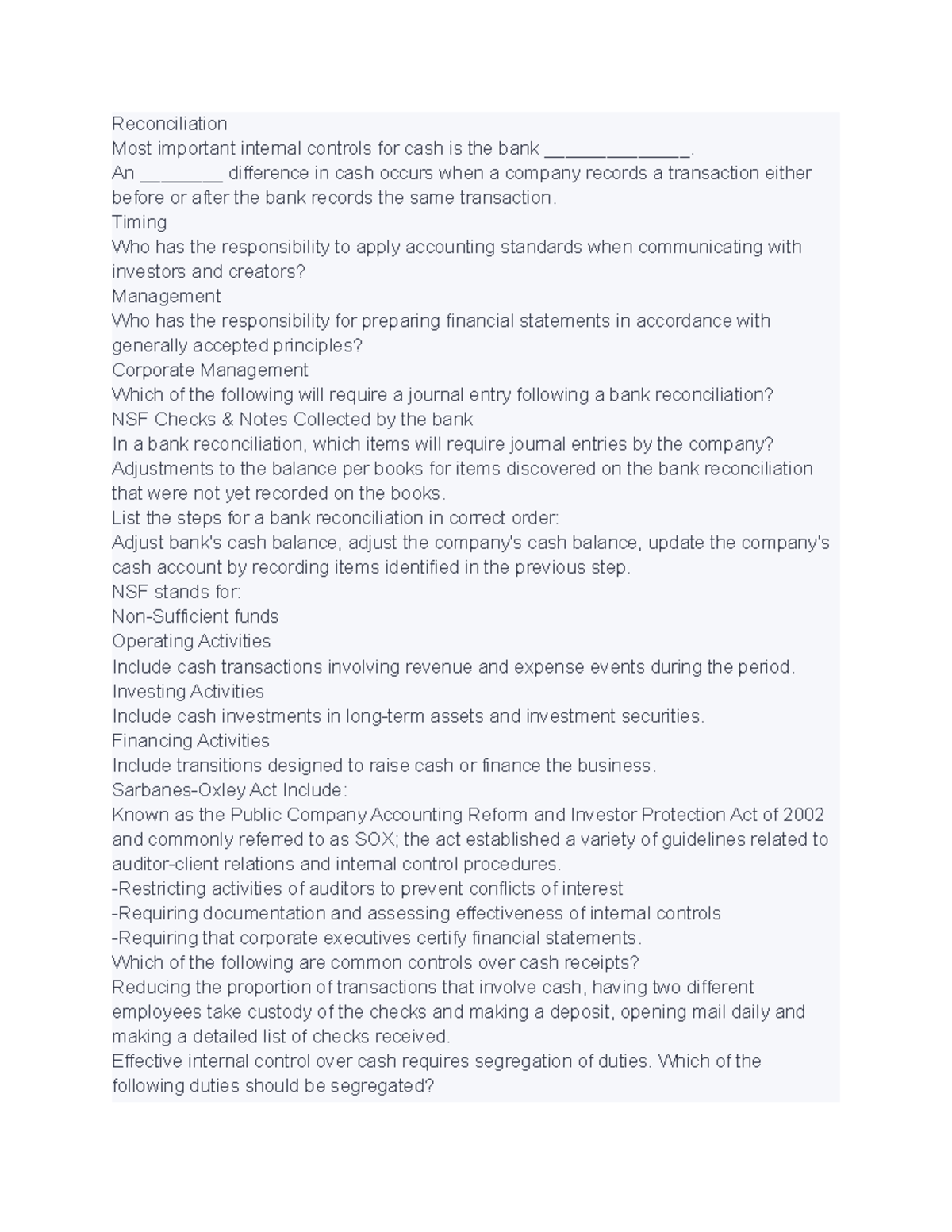**Detailed Caption:**

This image illustrates the importance of bank reconciliation and internal controls in the management of cash within a company. Key factors include the timing differences in recording transactions between the company and the bank, which often lead to discrepancies. Tammy, who oversees cash applications and communication within the organization, ensures that internal controls are maintained. Effective management necessitates understanding which transactions require journal entries following a bank reconciliation, such as sub-checks and notes collected by the bank.

The process of bank reconciliation involves several meticulous steps: 
1. Adjusting the bank's cash balance to reflect items like outstanding checks and deposits in transit.
2. Adjusting the company's cash balance for any discrepancies identified, ensuring accurate income recording.

Additionally, detailed analysis of funds includes cash transfers related to uncertain revenue and expense periods, encompassing cash investments, long-term assets, and associated financing activities.

The Sarbanes-Oxley Act (SOX) of 2002 is highlighted within this context. Known formally as the Public Company Accounting Reform and Investor Protection Act of 2002, SOX was implemented to increase transparency in financial reporting and establish stronger internal controls.

This image serves as a testament to the rigorous process of bank reconciliation, emphasizing the importance of detailed and accurate financial management practices.